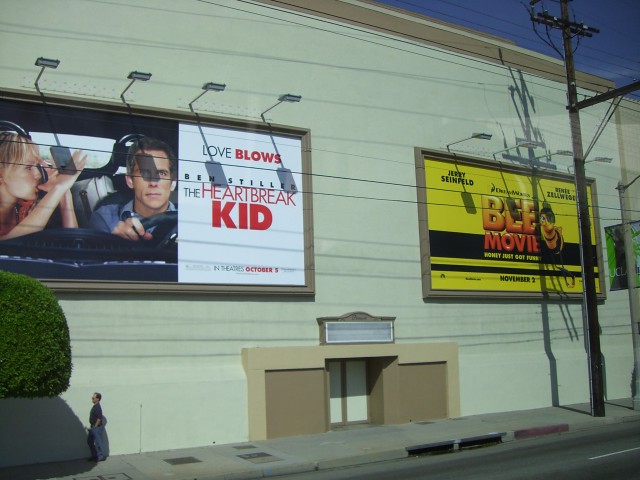This photograph captures the side of a building, likely a studio, adorned with multiple billboards. Despite the daytime setting, these billboards are equipped with lights to illuminate them at night, suggesting the studio uses them continuously to promote their movies. One prominent billboard advertises the movie "The Heartbreak Kid," featuring the tagline "Love Blows," and mentions an October 3rd release date. The billboard displays a large image of Ben Stiller behind the steering wheel of a car, with an unidentified woman next to him. Above the movie title, "The Heartbreak Kid," is Ben Stiller's name in bold letters. To the right, another billboard promotes "Bee Movie," which stars Jerry Seinfeld. This promotional poster also adds to the vibrant and dynamic façade of the studio building.